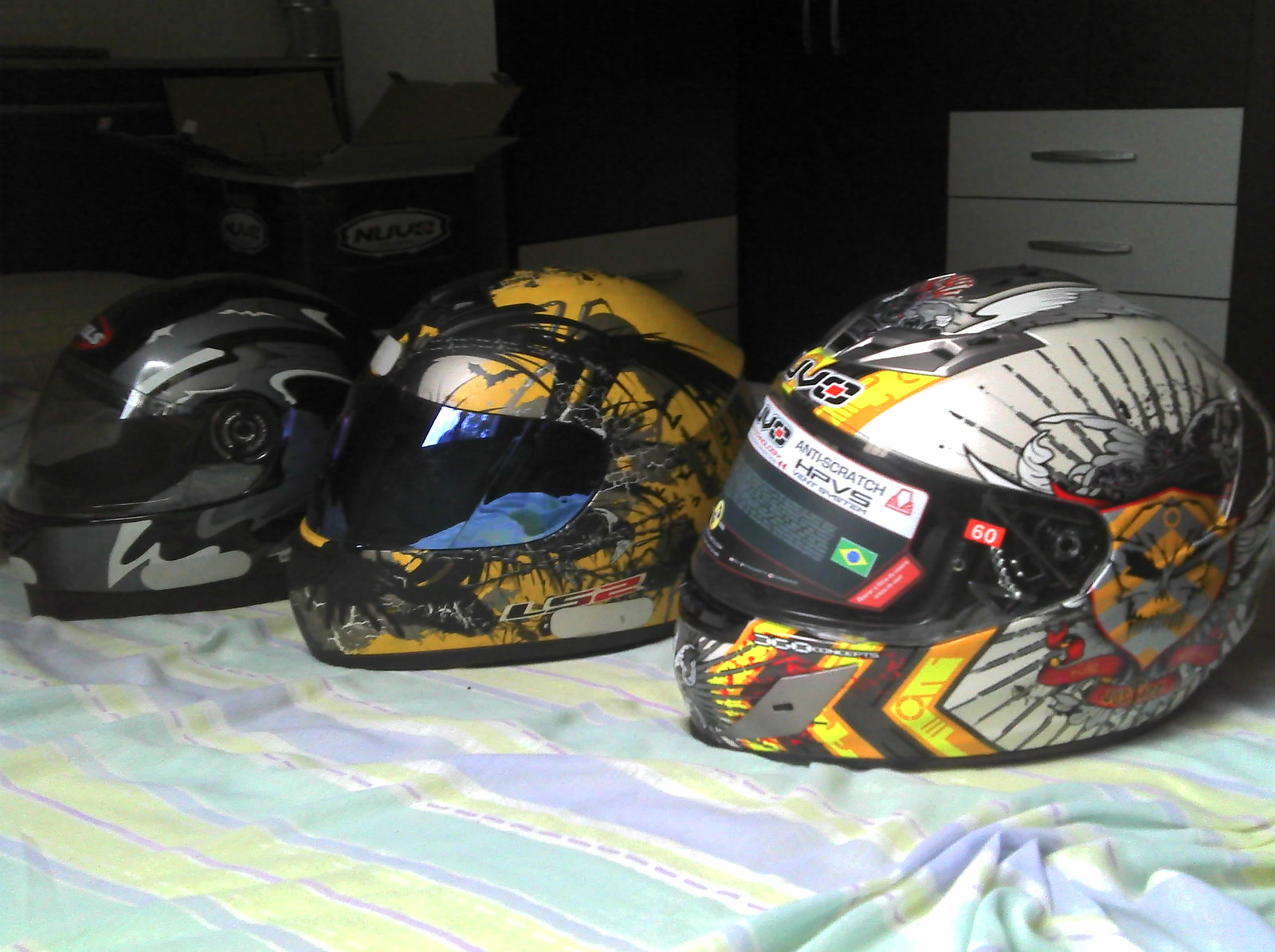The image is a color photograph taken in a bedroom. In the foreground, three motorcycle helmets are neatly arranged side by side on a crinkled blue and white striped sheet. Each helmet features a closed visor and distinct, unique designs: the helmet closest to us is adorned with an evil face motif in yellow, black, white, grey, and some orange, with the label "HPVS" at the top of the visor. The middle helmet showcases a light orange and black paint-splatter design, marked with the label "US2" under the face shield. The far-left helmet displays a grey and white camouflage pattern reminiscent of military fatigues. In the back right of the room stands a white dresser with long silver handles on the drawers, and a black wall behind it adds contrast to the scene. Additionally, some boxes, one labeled "NUUS," are faintly visible, complementing the cozy yet organized setting.